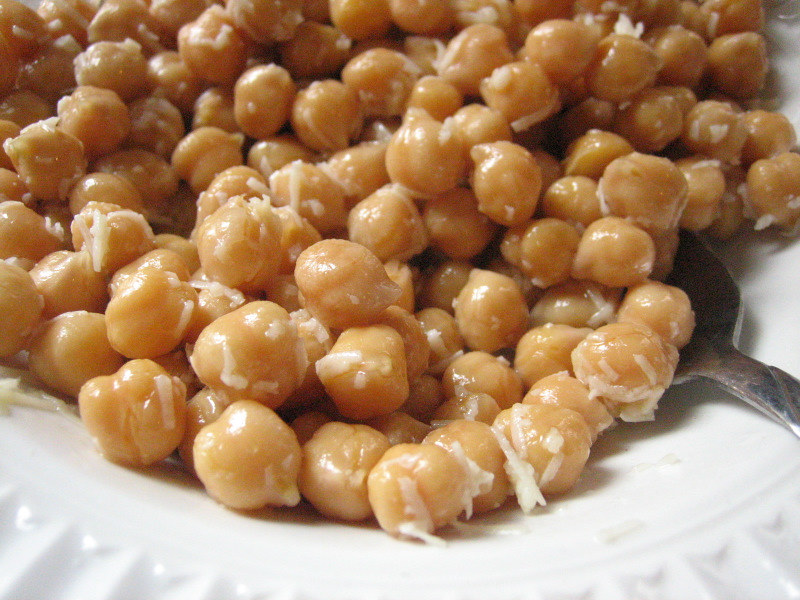An ornate round china plate, slightly visible at the edges, holds a generous serving of gleaming, cooked chickpeas (also known as garbanzo beans). The beans, making up the majority of the image, are bathed in olive oil and adorned with finely grated Parmesan cheese, which gives a whitish-yellow hue with reflective highlights suggesting a fresh, appealing coating. A partially visible utensil, likely a spoon based on its edge, peeks from underneath the chickpeas, adding a touch of casual readiness to the scene. The chickpeas, glossy and enticing, appear to be coated in a savory sauce, possibly mistaken for a sweet glaze in the overlapping interpretations. The overall imagery exudes a delicious invitation, enhanced by the elegant, rippled pattern of the decorative china plate peeking through.